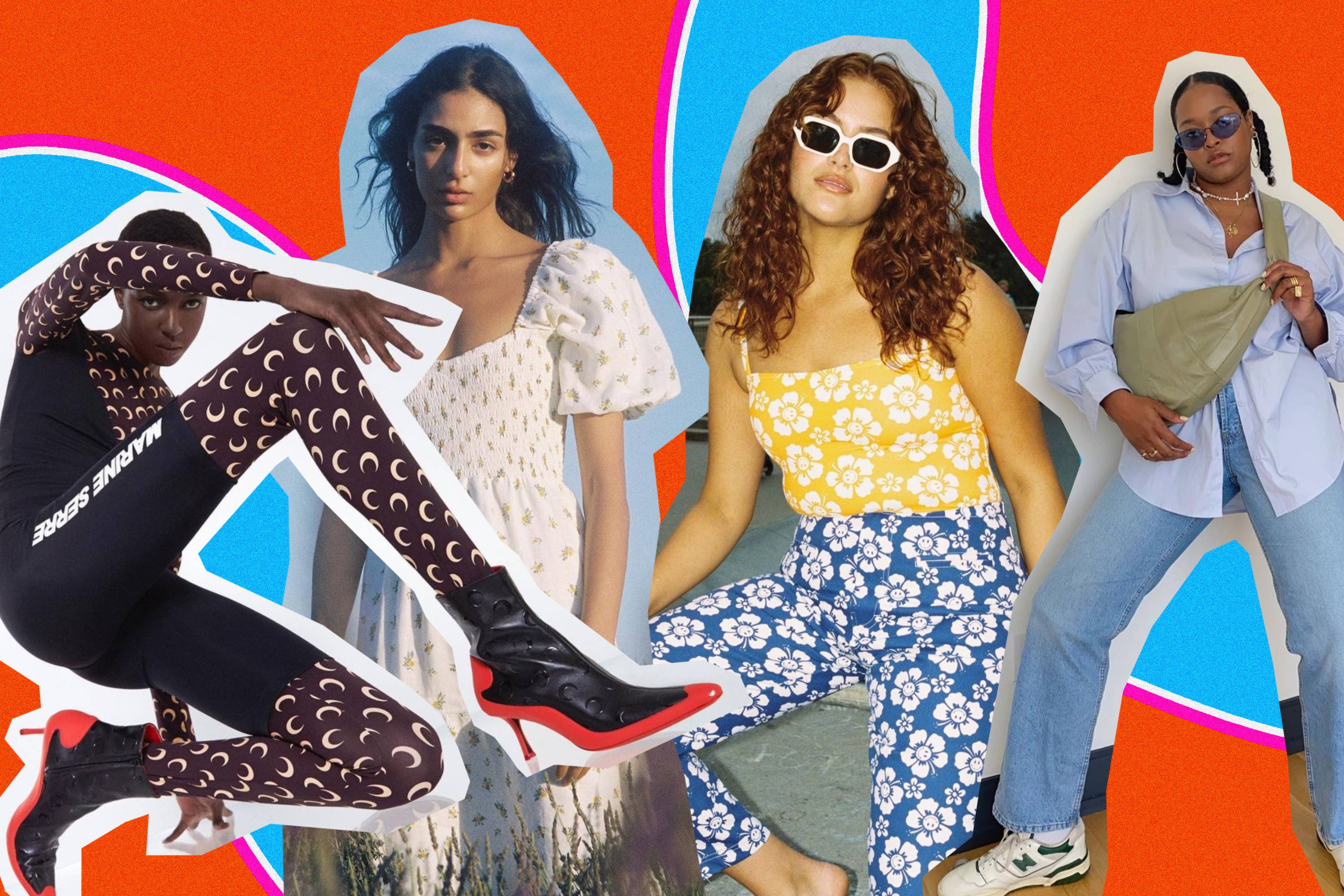This image showcases a set of four fashionable young women, positioned against a vibrant, multicolored red and blue rectangular background. From left to right:

- The first woman, a slender model with dark skin, is dressed in an intricate black suit adorned with white crescent moon patterns on the chest, sleeves, and stockings. Her ensemble includes striking black leather high-heeled boots that feature bright orange soles.
- Next is a young woman with long, flowing dark hair, wearing a simple yet elegant white sundress speckled with small dots.
- The third lady has curly red hair and sports white-rimmed glasses. Her outfit consists of a cheerful yellow top decorated with white flowers and blue pants that mirror the same floral pattern.
- On the far right stands a young woman exuding a more casual vibe. She has her hair styled in ponytails and is dressed in a light blue, buttoned-down shirt left open at the collar, paired with jeans and white tennis shoes. She carries a tan purse and wears a subtle necklace.

This ensemble of diverse styles against a striking background highlights each woman’s unique fashion sense.